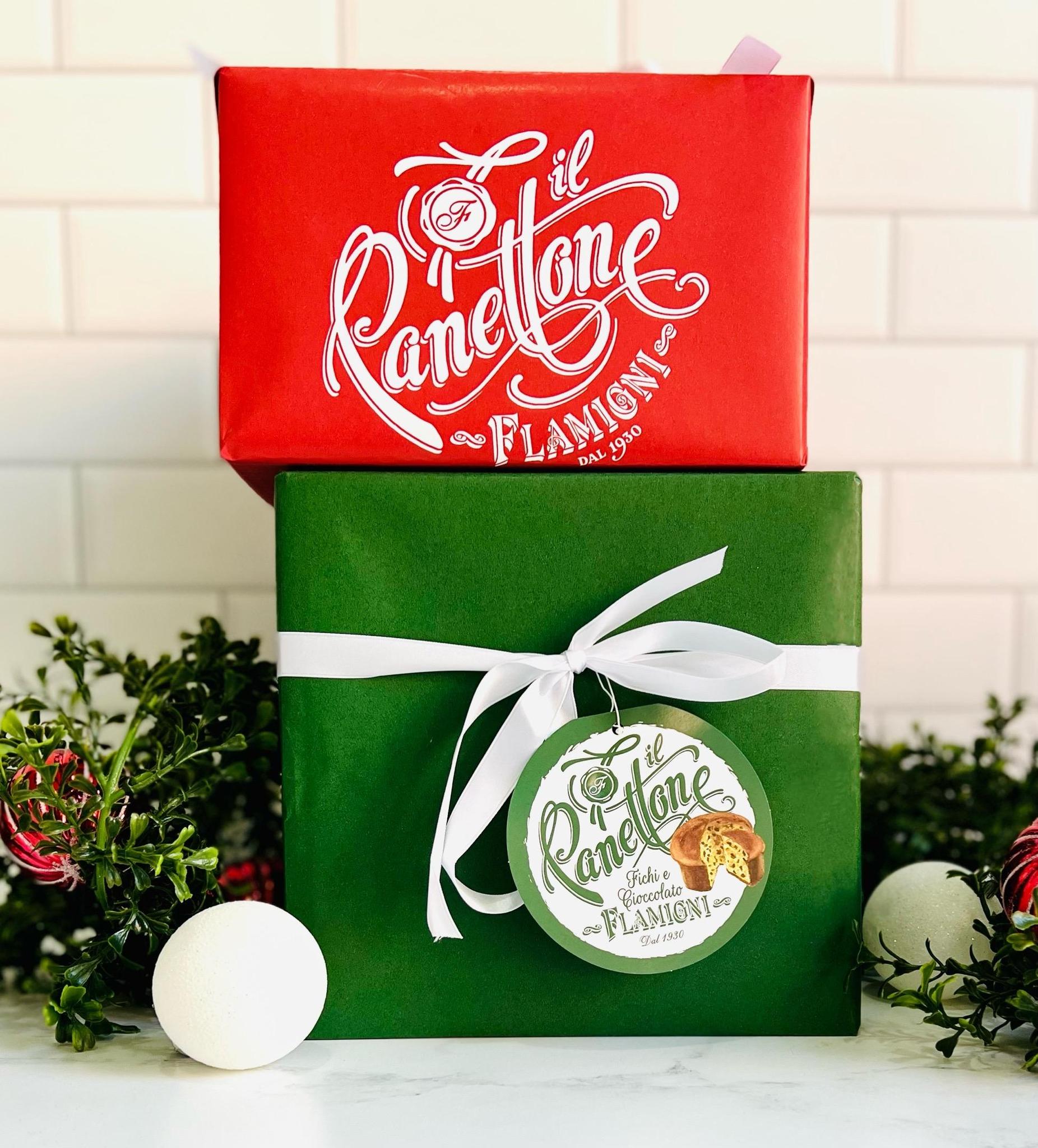In this vibrant photograph, there are two neatly wrapped presents stacked atop each other against a pristine white brick wall. The bottom gift is a green square box adorned with a white ribbon tied into a bow. Attached to its ribbon is a green-bordered circular label depicting an image of a sliced loaf of bread, with the inscription "Panettone Ficci e Cioccolato Flamigni" in green Italian cursive. Resting on top is a slightly smaller red square box, also wrapped meticulously, bearing a label that reads "Panettone Flamigni D.A.L. 1930" in elegant white cursive. Both boxes suggestively contain Italian cakes, a Panettone, a traditional festive dessert. Surrounding the presents is a lush arrangement of green holly-like leaves and two white decorative balls, creating a festive atmosphere. The scene is set on a clean, white shelf, enhancing the overall crisp and celebratory aesthetic.